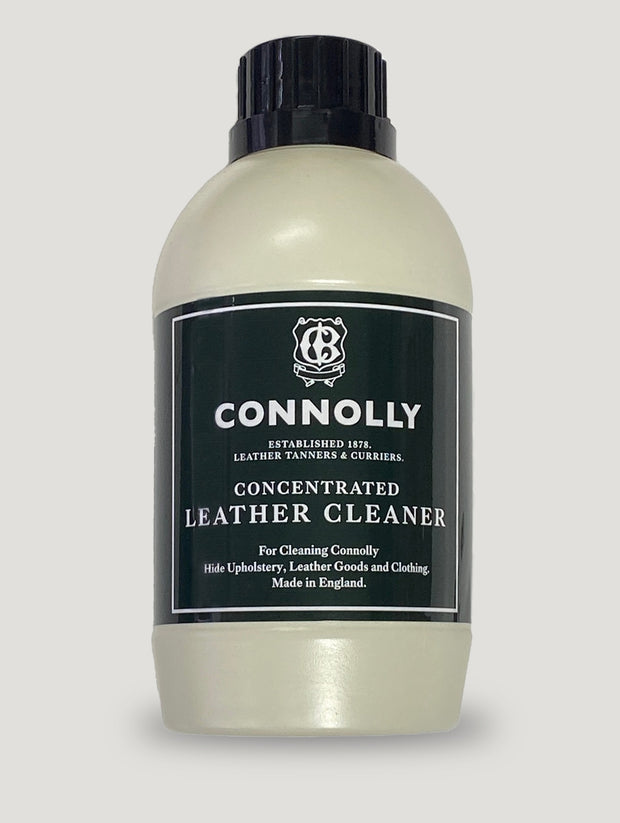The image features a small opaque white bottle with a black twist-off plastic cap, standing against a light grayish white background. The bottle boasts a prominent, dark label encircling its midsection, which appears either in black or very dark green. Central to the label is a bold white rectangle with a delicately thin border. At the heart of this rectangle lies a shield emblem bearing an initial. Below the emblem, the label presents the text "Connolly" in bold white lettering, followed by "Established 1878 Leather Tanners and Curriers." Additional text below reads, "Concentrated Leather Cleaner for Cleaning Connolly Hide Upholstery, Leather Goods, and Clothing." The label concludes with "Made in England." This meticulous detailing emphasizes both the historical prestige and the specific use of the product.